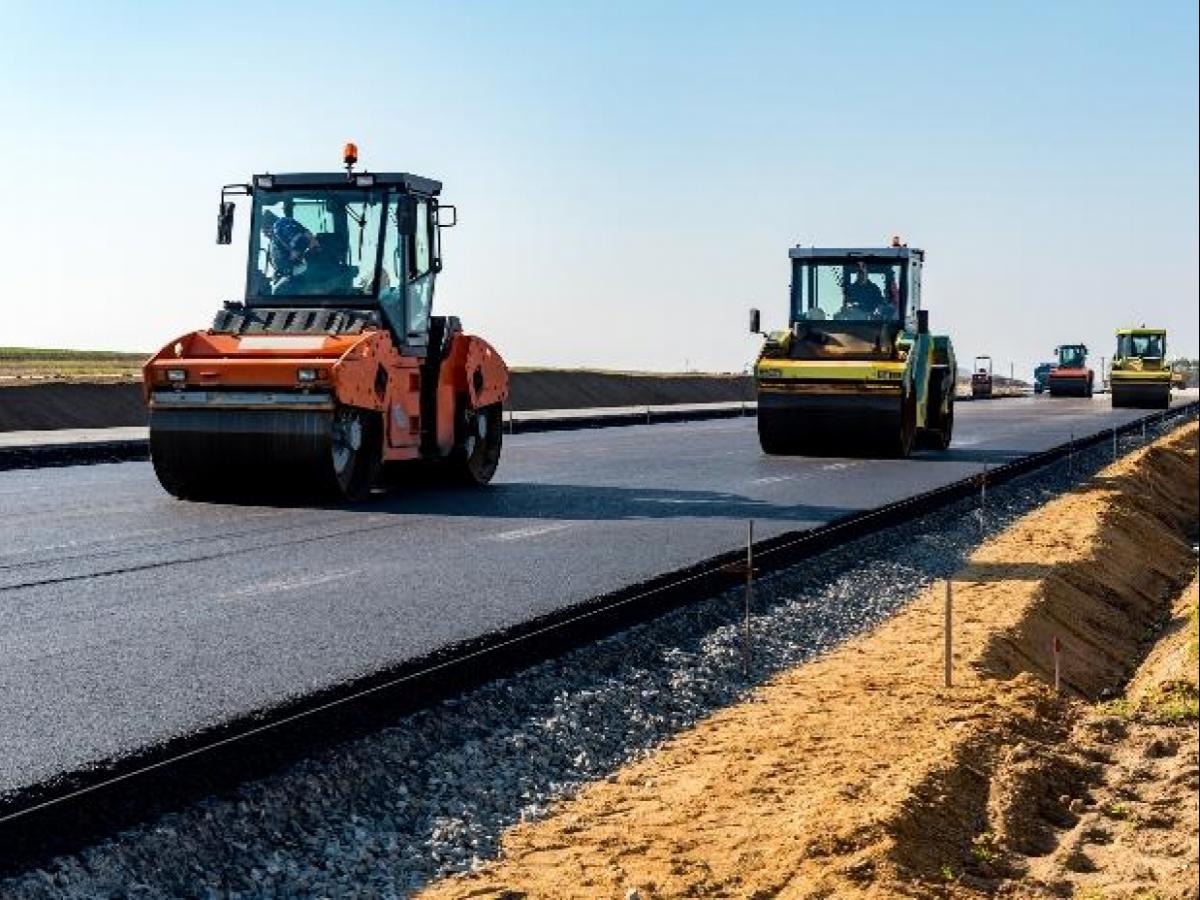This daytime color photograph vividly captures a fleet of construction vehicles working meticulously on a newly-paved black asphalt road. The composition features multiple steam rollers of varying colors—two orange and two yellow—each equipped with large black rollers at both the front and rear. The lead vehicle, an orange roller, is followed closely by a yellow one and further back, other vehicles can be seen. These vehicles, relatively small trucks with substantial rollers, are methodically flattening the fresh pavement. The drivers are visible within their glass-enclosed compartments, with one in the foreground noticeably leaning out the side window, peering behind.

The freshly asphalted road begins on the right and stretches diagonally to the lower left. Adjacent to the road on the right lies a mound of light brown dirt, punctuated by small sticks, while a band of gravel runs along the upper right. To the left, a raised flat area covered in grass and soil is visible, contrasting with the road's dark hue. In the background, beyond the mound, another strip of black asphalt can be seen. The sky above is partly blue with a light white haze, casting a diffuse glow over the bustling scene.